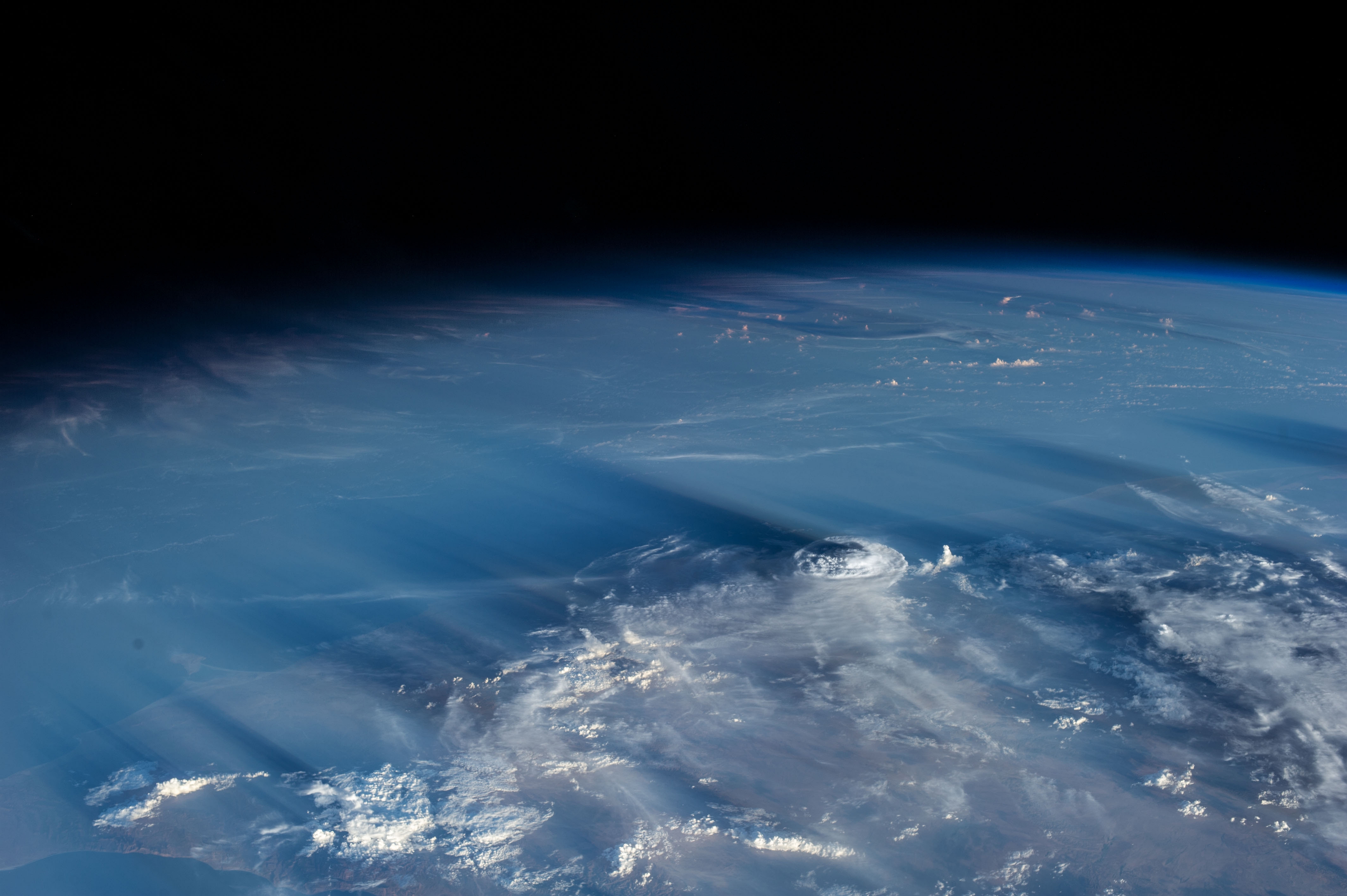The image shows a striking view of a planet from space, likely Earth, characterized by its almost alien appearance. The top one-fourth of the picture is pitch black, representing the void of space. Below, the curvature of the blue planet emerges prominently, adorned with wispy clouds. The notable feature is a possible mountain poking above the atmosphere, though it might also be a dense cloud formation resembling a hurricane. The bottom third of the image includes white areas that could signify clouds, ice, or snow, contributing to the planet's chilly and wintry aspect. Light from an unseen source in the bottom right-hand corner casts diagonal shadows across the scene. The picture appears to be a zoomed-in view, suggesting it might be capturing vast oceanic expanses with possible waves or landmasses, although the image is partially cut off, making detailed identification challenging. The overall impression is of a cold, blue, and uniquely detailed planetary surface as seen from a high vantage point in space.